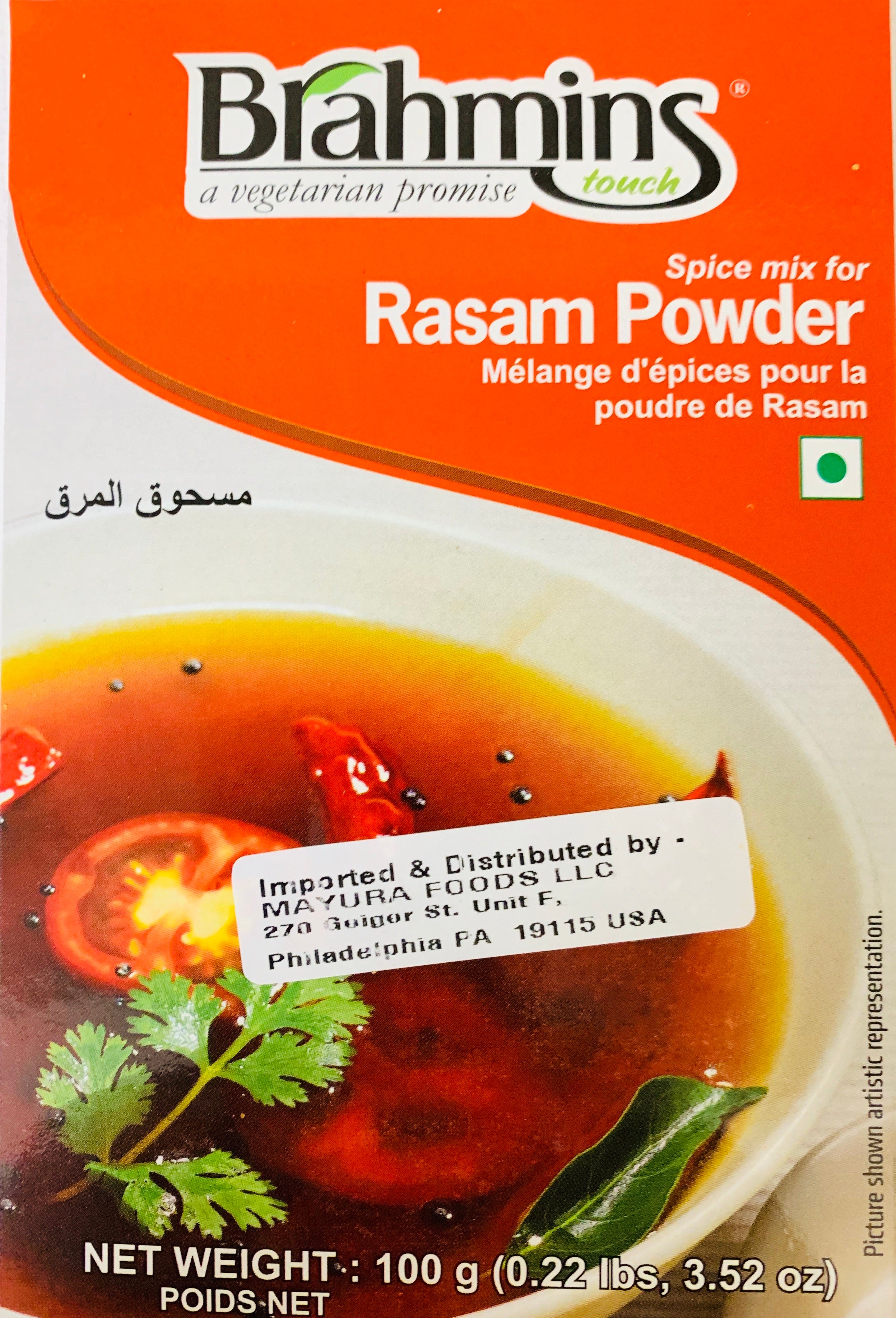The image depicts the front of a food product box named "Brahmins," branded with "A Vegetarian Promise." The top half of the box features a bold red color and is dominated by the text "Brahmins" or "Brahman's Touch" alongside a large orange swirl. To the right, it states "Spice Mix for Rasam" with a French translation, "Mélange de pisse pour la poudre de rasam." Below this, we see a detailed photograph of a white bowl filled with a clear broth, likely rasam, garnished with cherry tomatoes, chilies, cilantro, parsley, and whole leaves. The broth appears either brown or red. There's additional text in another alphabet at the top of the bowl. On the package, a green-outlined small square with a centered green dot is visible, along with an importer’s sticker reading "Imported and Distributed by Mayura Foods, LLC, 278 Philadelphia, Pennsylvania 9115 USA." Alongside, it lists the net weight as “100 grams (0.22 pounds, 3.52 ounces)” and includes a disclaimer that the picture is an artistic representation. The overall background of the box is primarily white with an emphasis on the detailed, vibrant imagery of the soup and clear product labeling.